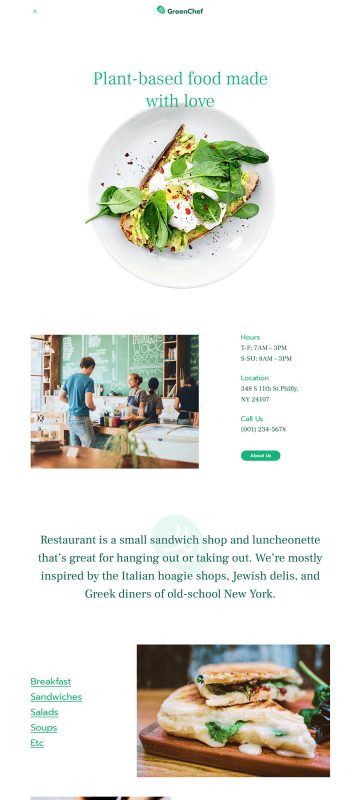In this promotional image for Green Chef, prominently displayed in the top center is the website's name and logo, both in a vibrant green color. Beneath the logo are the words "Plant-Based Food Made with Love." Below this tagline is a visually appealing image of a dish served on a white plate. The dish appears to be a triangular pastry, possibly made from dough, topped with an egg and garnished with fresh vegetable leaves. Scattered around the plate are small black dots, likely indicating the presence of pepper or another type of seasoning. 

Directly underneath this, a squared box contains another image depicting a scene from within the restaurant. A woman, presumably a cashier, is at the register, engaged with a man who is about to place an order. Both individuals are white, and in the background, two more women can be seen working behind the counter. 

To the right of this image, there are three informational sections labeled "Hours," "Locations," and "Call Us." The hours of operation are listed as Tuesday through Friday from 7 a.m. to 3 p.m., and Saturday through Sunday from 8 a.m. to 3 p.m. The location is specified as 348 South 11th Street, South Philly, New York, 24107.